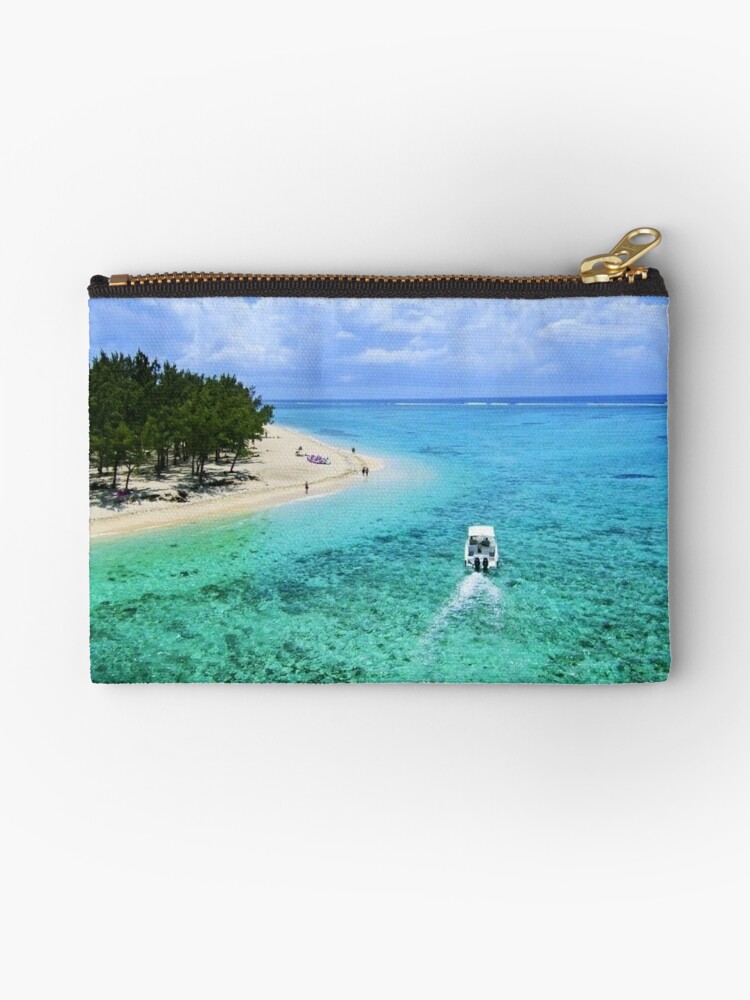This image showcases a rectangular wallet or pouch set against a gray background. The wallet features a prominent gold-colored zipper at the top. The artwork on the wallet beautifully depicts a tropical beach scene. On the left side, green trees are growing on the sandy shore. The beach, lined with tan-colored sand, has several people walking along its length. In the middle of the scene is a white boat gliding through the clear, light green ocean waters. Above the beach, the sky is filled with white clouds. The entire scene exudes a calm and tropical vibe, capturing a serene moment by the sea.